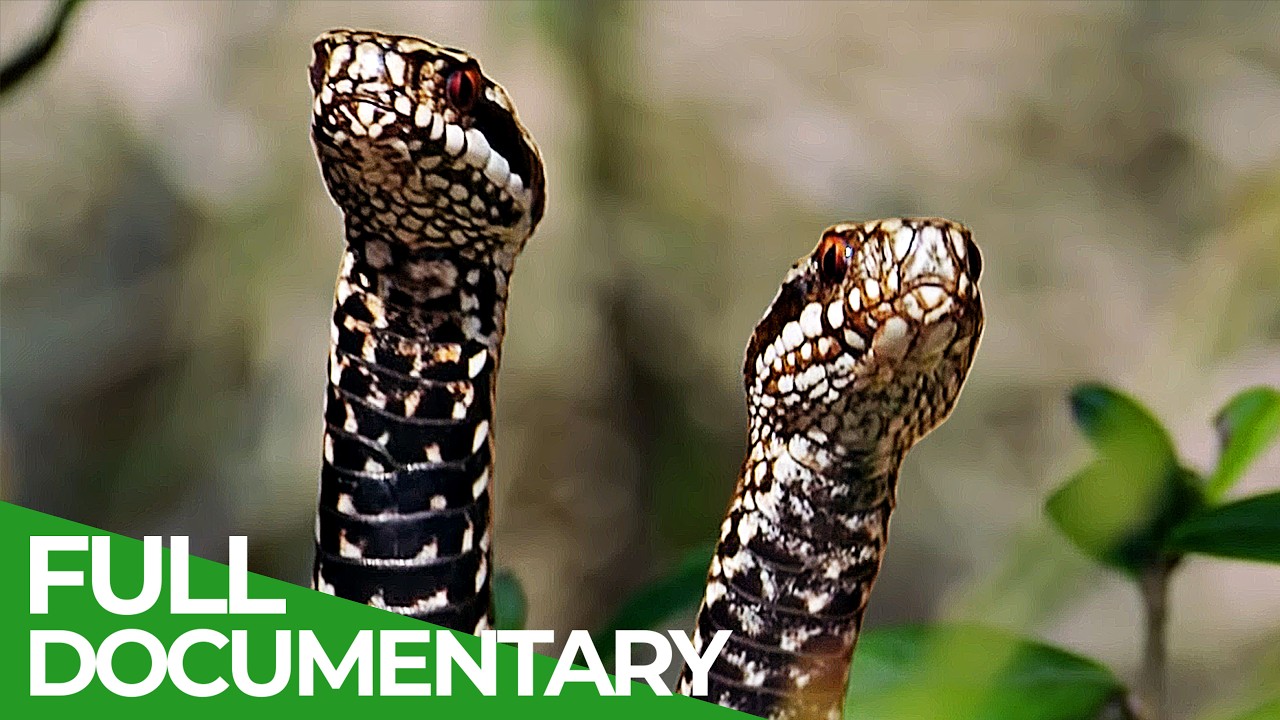This image appears to be a title screen from a documentary. The central focus is a large brown bear, positioned slightly to the left of the center, walking on all fours through a grassy field dotted with white flowers. The bear is framed by the lower portions of two thin tree trunks in the foreground, each with sparse limbs hanging down. In the blurred background, a dense forest of green trees stretches out, enhancing the wilderness ambiance. The grassy field shows a yellowish tint, possibly suggesting a late afternoon or sunset setting. In the bottom left corner, a green triangle with bold, white text prominently displays "full documentary." The photograph is rectangular, with its length prominent along the top and bottom sides. The bear's direct and intense gaze towards the camera adds a compelling and dynamic element to the scene.